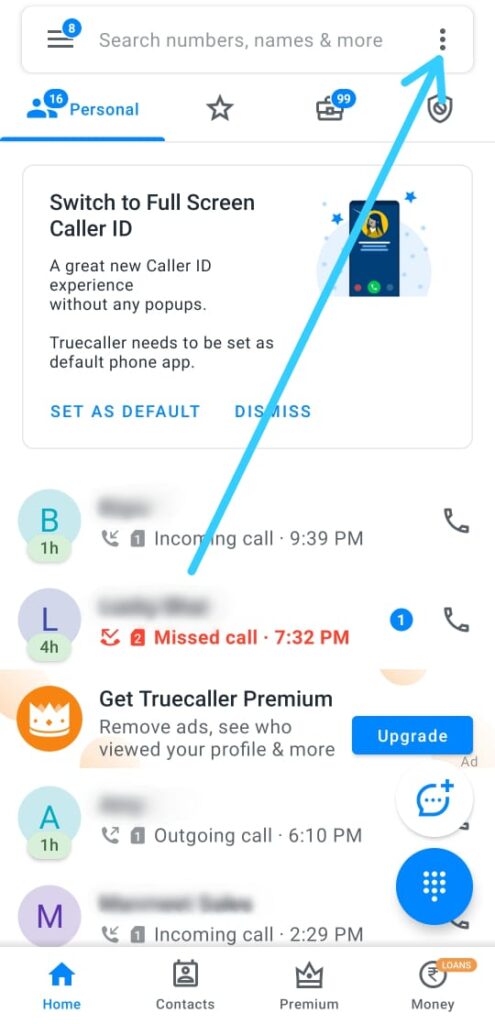The image depicts a screenshot taken on a cell phone showing an interface of a particular app. At the top, there is a search bar with various functional icons and options. Notably, the search bar contains three horizontal stacked lines in black, accompanied by a blue notification bubble with the number '8' in white ink. 

Displayed within the search bar is the prompt "Search numbers, names, and more..." in gray text. Adjacent to this prompt, a vertical ellipsis (three vertically aligned dots) appears, suggesting additional options. A blue arrow is pointing to this ellipsis, indicating its importance or next step action.

Below the search bar, the interface features several categorized buttons labeled "Personnel," "Favorites," and "Cats." Additionally, there's text instructing users about switching to full-screen Caller ID and creating a new Caller ID experience, specifying: "Truecaller needs to be set as the default phone app."

Further down, the screenshot reveals a call log showing recent call activity, including calls that were missed. However, the names of the callers have been obscured, ensuring privacy by scratching out the identifying information.